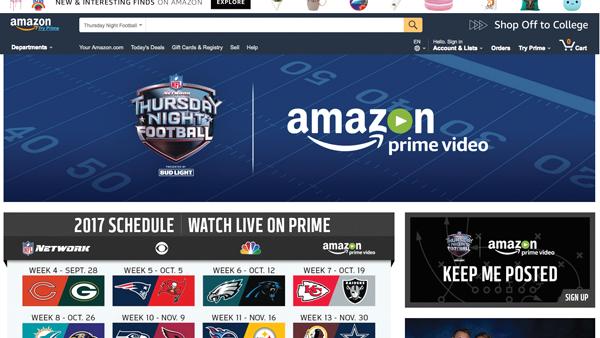The image is a detailed screenshot of the Amazon homepage, prominently featuring their Thursday Night Football promotions. In the top left corner, the Amazon logo is visible, adjacent to a large search bar displaying the text "Thursday Night Football." On the top right of the page, there is a link labeled "Shop Off to College."

Dominating the center of the page is an expansive image of a football field, showcasing the yard lines from the 20 to the 50 in one direction, and the 40 in the opposite direction. Superimposed on the field is the logo for "Thursday Night Football on ABC," with "Amazon Prime Video" text spanning across the image. To the left, the tagline "2017 Schedule. Watch live on Prime. NFL Network" is visible, accompanied by the logos of CBS, NBC, and Amazon Prime Video.

Below this, the partial football schedule is displayed. It lists:
- **Week 4**: September 28, featuring Chicago vs. Green Bay,
- **Week 5**: October 5, featuring New England Patriots vs. Tampa Bay Buccaneers,
- **Week 6**: October 12, featuring Philadelphia Eagles vs. Carolina Panthers,
- **Week 7**: October 19, featuring Kansas City Chiefs vs. Oakland Raiders.

Future weeks and their corresponding teams are hinted at but the image is cut off before the full schedule is shown.

On the right side, the Amazon Prime Video logo appears alongside the prompt "Keep Me Posted" with a "Sign Up" button situated below.